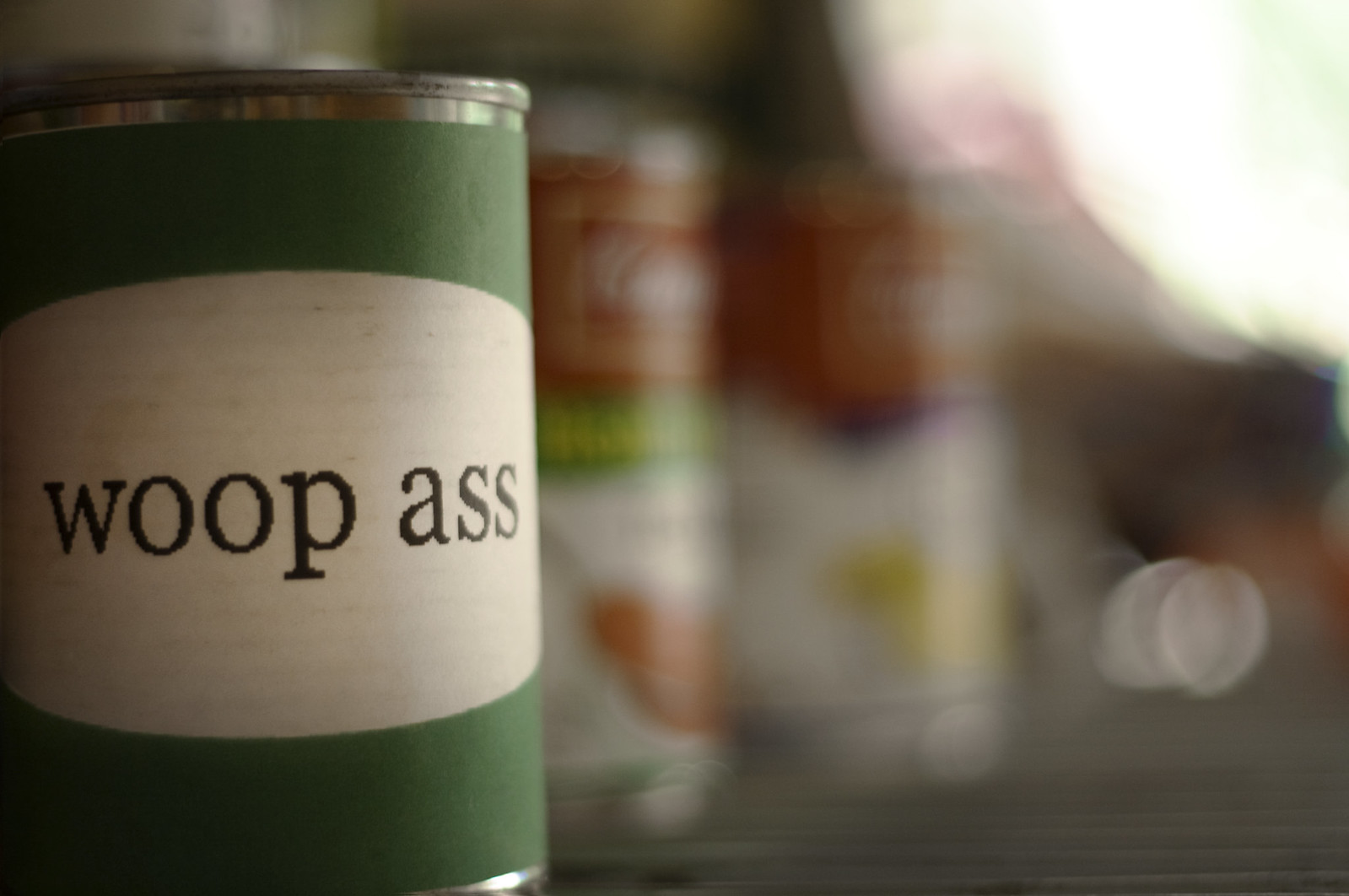A well-organized image features a neatly arranged row of various colored cans on a shelf. The can closest to the viewer stands out with its green and white design, prominently displaying "WUPAS" in bold black lettering. The cans behind it create a vibrant, albeit blurry, backdrop, flaunting a range of colors including orange, red, white, and green. Towards the far end of the row, slightly beyond the third can, a white plastic-capped tube lies on its side, adding a distinct element to the composition. The primary focus remains on the sharply detailed silver can in the foreground, while the rest of the items gradually blur into the background, offering a sense of depth and perspective to the scene.